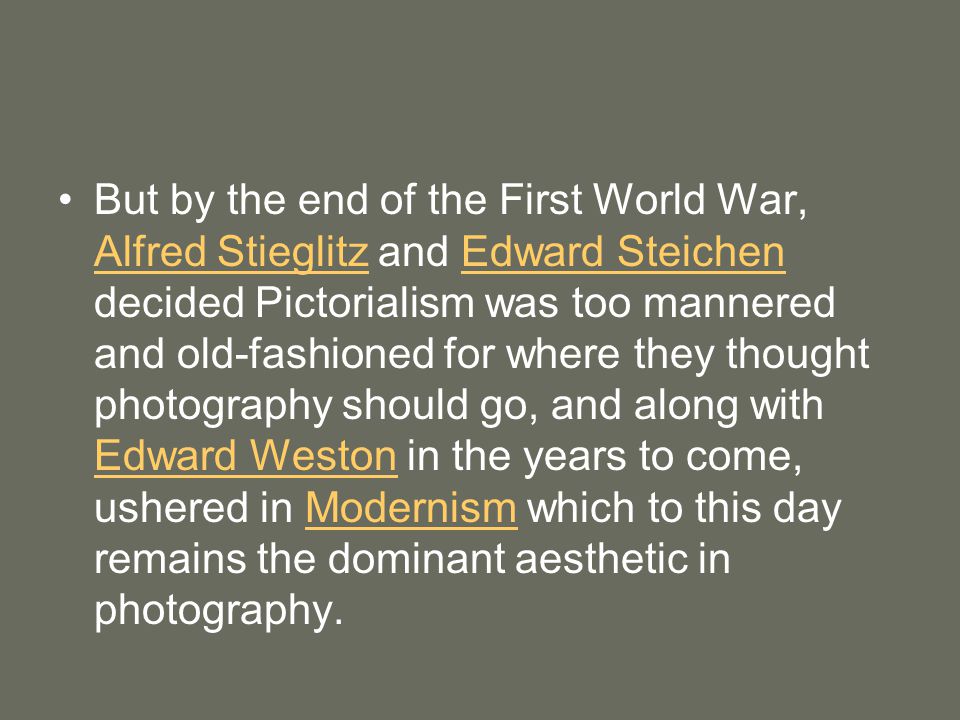The image features a neutral, gray rectangular background with centrally positioned text, resembling a PowerPoint slide. The text, which is predominantly white, begins with a small white bullet point on the left. It conveys historical information about the evolution of photography, stating: "But by the end of the First World War, Alfred Stieglitz and Edward Steichen decided pictorialism was too mannered and old-fashioned for where they thought photography should go. And along with Edward Weston, in the years to come, ushered in modernism, which to this day remains the dominant aesthetic in photography." Notably, the names "Alfred Stieglitz," "Edward Steichen," and "Edward Weston" are highlighted in yellow and underlined, as is the term "modernism." The image's clean and straightforward design, with its large, easy-to-read text, is well-suited for educational purposes.